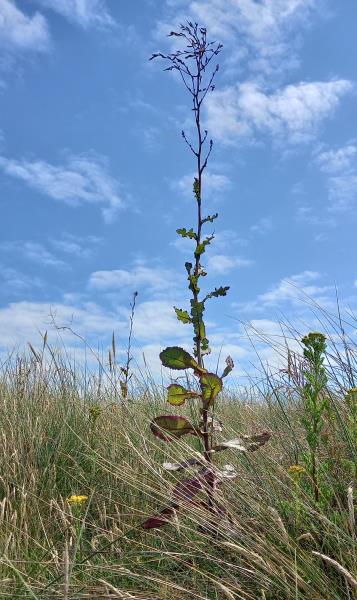The image depicts a serene outdoor scene with a predominantly blue sky, scattered with wispy white and gray clouds. Dominating the foreground is a tall, lanky plant with a mix of green and red leaves, extending upwards from a field of diverse vegetation. The plant's lower leaves are broader, gradually becoming smaller higher up, where it branches out into small buds, slightly silhouetted against the sky. Surrounding this central plant, the ground is covered in various types of grass, some of it appearing dried and white. To the left and right, clusters of small yellow flowers punctuate the landscape, along with other green plants and dried weeds typical of a marsh-like area. The sunlight reflects off the plant leaves and grass, illuminating the field and enhancing the tranquil atmosphere of the scene.